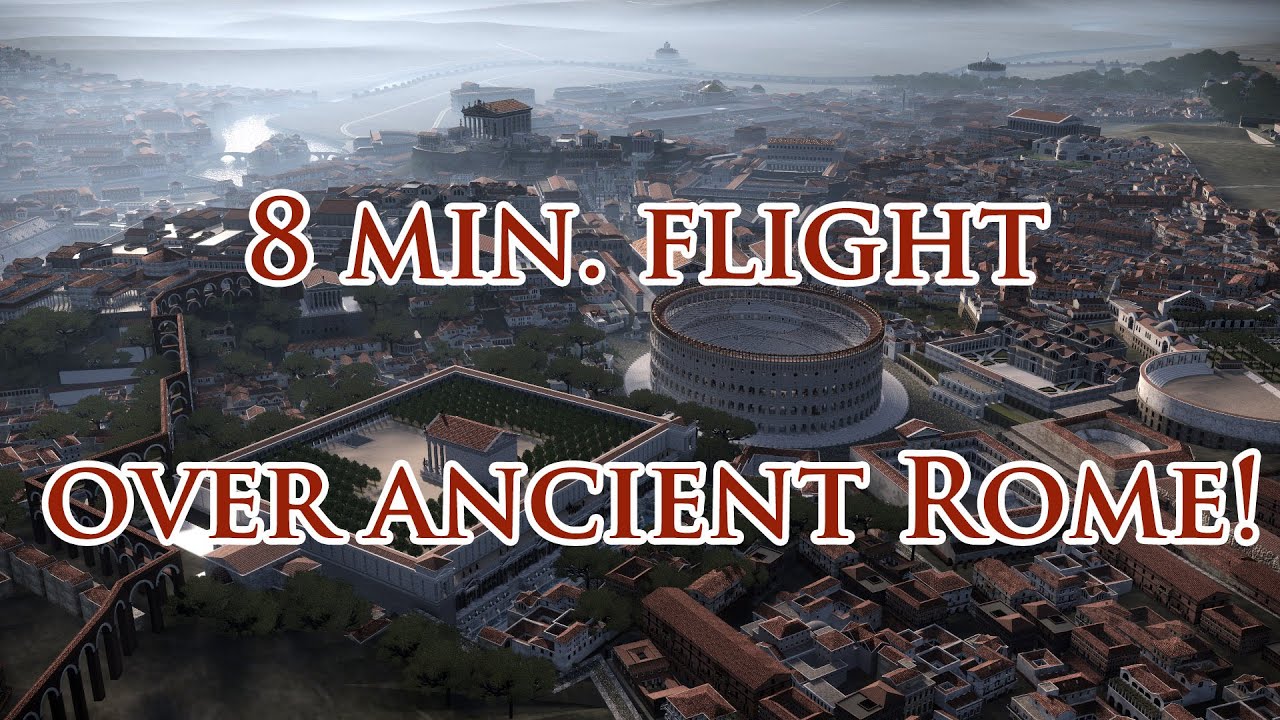The image, likely a YouTube thumbnail or an advertising poster, showcases a computer-generated, bird's eye view of ancient Rome in its prime. The vibrant and detailed animation appears to render a morning scene, casting a warm glow over the cityscape. The prominent red letters with a white outline boldly announce "8-minute flight over ancient Rome!" featuring an exclamation point for emphasis. The scene includes key landmarks like the fully intact Colosseum, the grandiose Circus Maximus, Caesar's Palace, and Palatine Hill. In the background, with a hint of mist adding mystique, one can see the Tiber River and the Seven Hills, offering a broad and immersive vista of the ancient metropolis. This captivating image advertises an eight-minute drone-like flight, possibly through real or CG means, over ancient Rome, inviting viewers to explore its historical splendor.